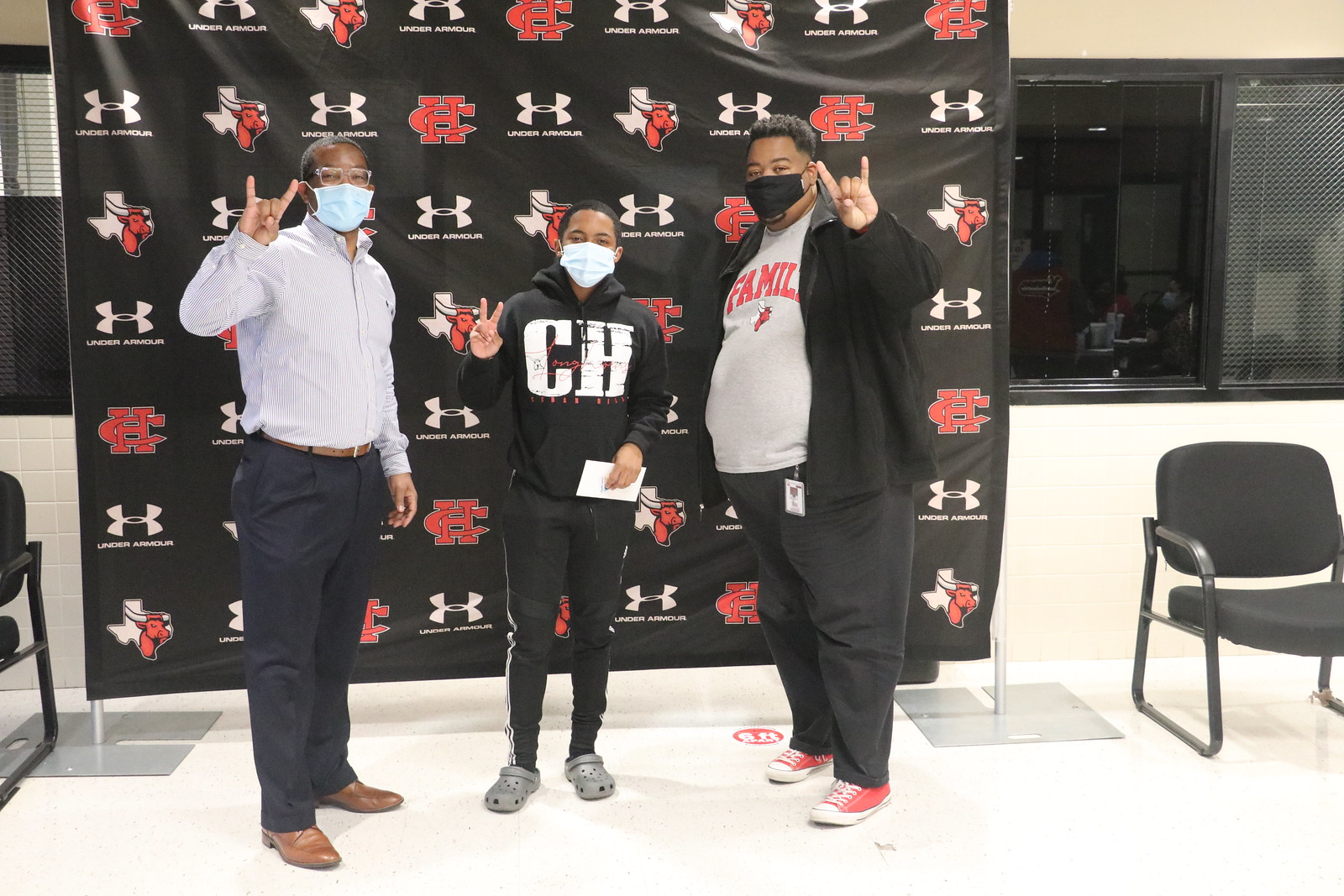In the image, three African American males are standing in front of a black banner adorned with white Under Armour and CH logos. On the left, a man with short gray hair and glasses is making a devil's horn gesture with his right hand while wearing a white button-down shirt, black pants, brown loafers, and a COVID-19 mask. The boy in the middle, sporting short dark hair, is dressed in a black hoodie with white "CH" text, black jeans, and gray Crocs while holding up a peace sign and also wearing a mask. The man on the right, slightly overweight, has on a gray sweater with red "family" text, a black coat, black pants, and red tennis shoes. All three individuals are wearing COVID-19 masks. The backdrop behind them features a black background with a prominent white Under Armour logo.